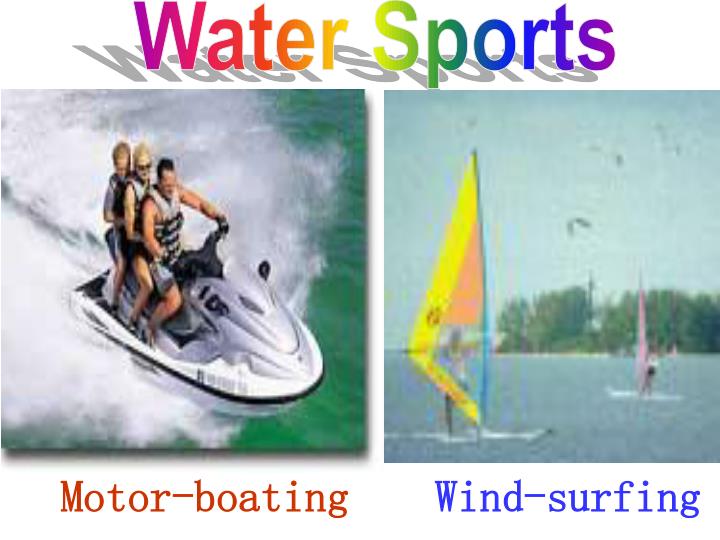A vibrant advertisement for a water sports company features a top-centered, colorful "Water Sports" title, transitioning through shades of the rainbow from purple and pink to blue and purple, accented with a light gray shadow that creates a striking depth effect. Below the title, the rectangular image is divided into two square photos. The left photo showcases three people on a white, gray, and silver jet ski gliding over the ocean's green waters; the caption beneath it, in red print, reads "Motor-Boating," though it's clearly jet skiing. The right photo captures an older-looking, dynamic scene of two individuals windsurfing with green and yellow sails against a backdrop of blue skies, ocean, and distant trees. The caption below it, in blue print, accurately describes "Wind-Surfing."